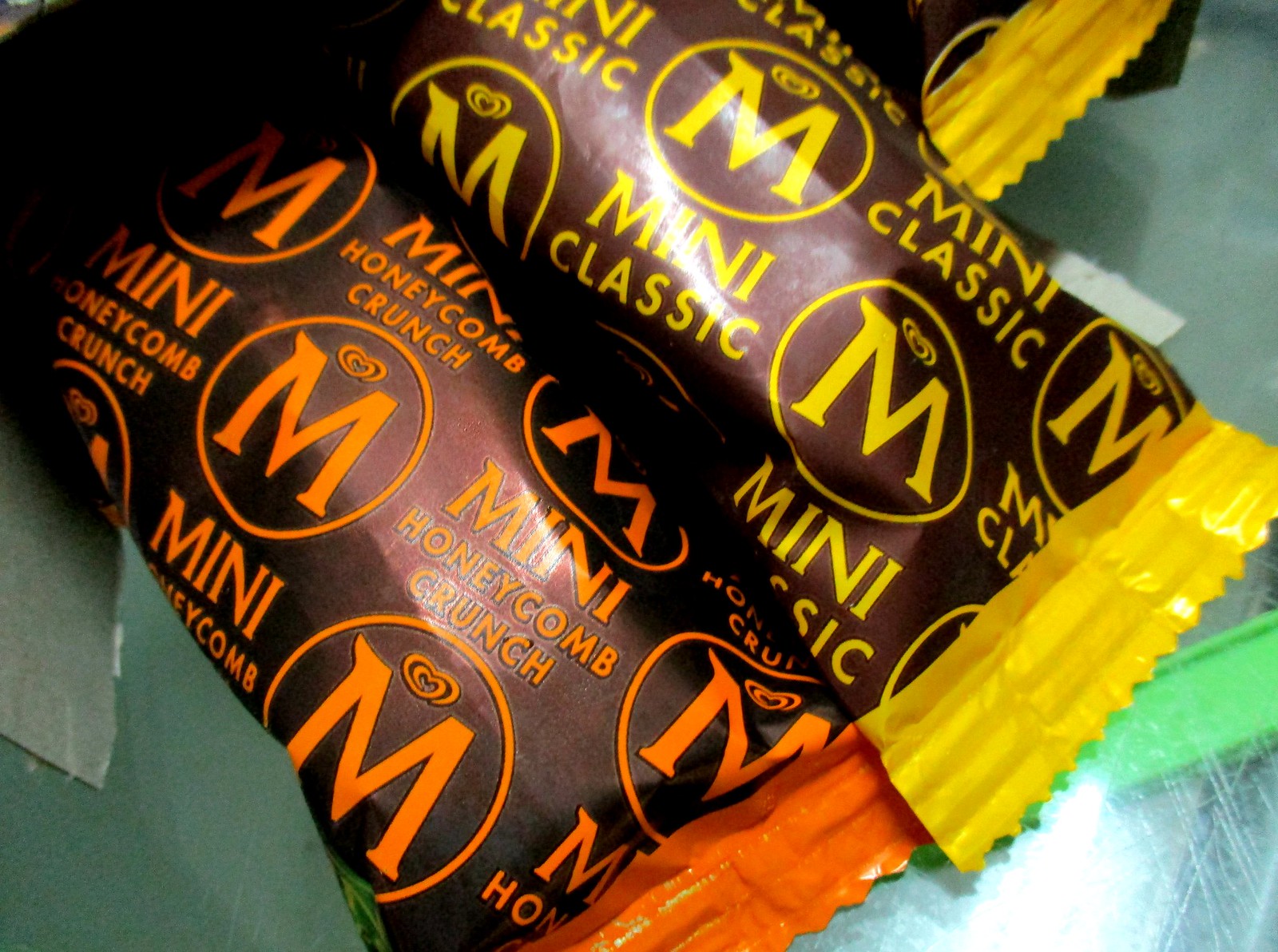This color photograph, taken in a landscape orientation as part of product photography, shows a close-up view of two different candy bars from a variety pack. The box is open, revealing the bars partially emerging from their packaging against a blurred, indistinguishable green background. Both candy bar wrappers share a brown base color but are distinguished by their accent colors: one features yellow accents and the other orange. The yellow-accented wrapper reads "Mini Classic," while the orange-accented one reads "Mini Honeycomb Crunch." Both wrappers feature an identical logo consisting of a large 'M' inside a circle, with a smaller heart and larger heart surrounding the letter. Yellow edges frame the Mini Classic bar's packaging, whereas the Mini Honeycomb Crunch has orange edges. Additionally, a part of a yellow snack is visible in the top right corner with text partially cut off. The photographic style is representational realism.